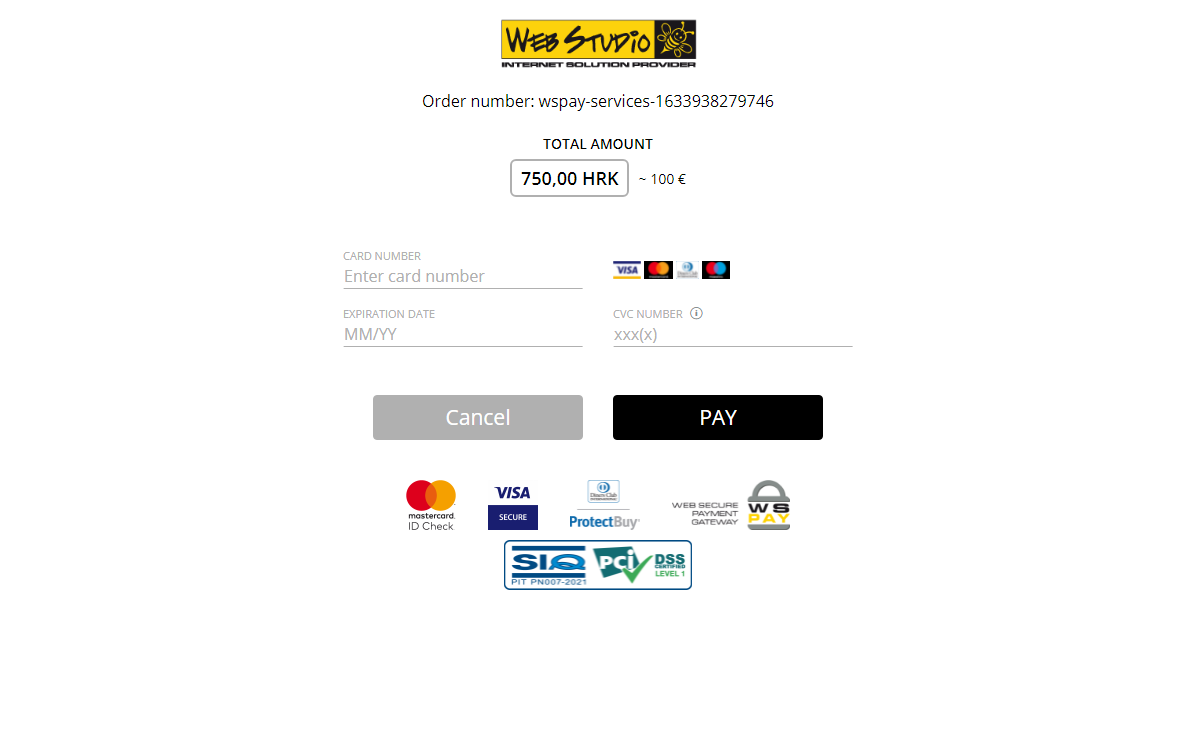This image displays a payment interface for WebStudio, an Internet Solution Provider, featuring their tagline prominently. The order number, "wspay-services-1633938279746," is specified, and the total amount is listed as 750,00 HRK, which is roughly equivalent to 100 euros. The payment section includes fields for entering the credit card number, expiration date, and CVC code, although these fields are currently empty. Below these fields are two buttons: a black "Pay" button and a gray "Cancel" button.

The interface showcases icons for various accepted payment methods, including Visa, MasterCard, Maestro, Diners Club International, as well as security logos such as MasterCard ID Check, Visa Secure, and others that suggest a secure payment process (Project Buy, Web Secure Payment Gateway, ISQ, PCI DSS Certified Level 1).

Despite the numerous security logos, which imply a high level of safety and certification for credit card transactions, the overall presentation may come across as excessive and potentially suspicious. However, the choice to proceed with the payment rests with the user.